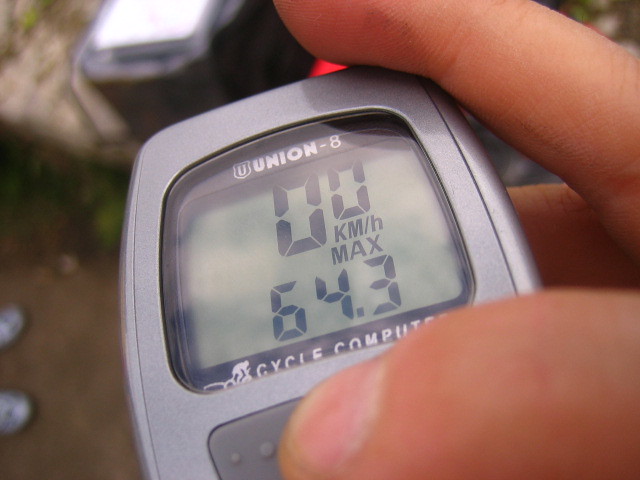A detailed close-up image of a cycle computer, which is a device that attaches to a bicycle to track distance and speed. The prominently displayed LCD screen indicates a current speed of "0 km/h" with digital, segmented numerals. Below this, the display shows a maximum recorded speed of "64.3 km/h" labeled with "MAX". The device is encased in a gray housing, and a thumb and forefinger are gripping it, hinting at a button beneath the thumb made from darker, rubberized material. The background is heavily blurred, featuring indistinguishable brown and gray shapes, suggesting varied elements. A faint red light is visible behind the forefinger, whose origin is unclear, and there's a hint of green, likely plants, implying the photo was taken outdoors, possibly near a vehicle.